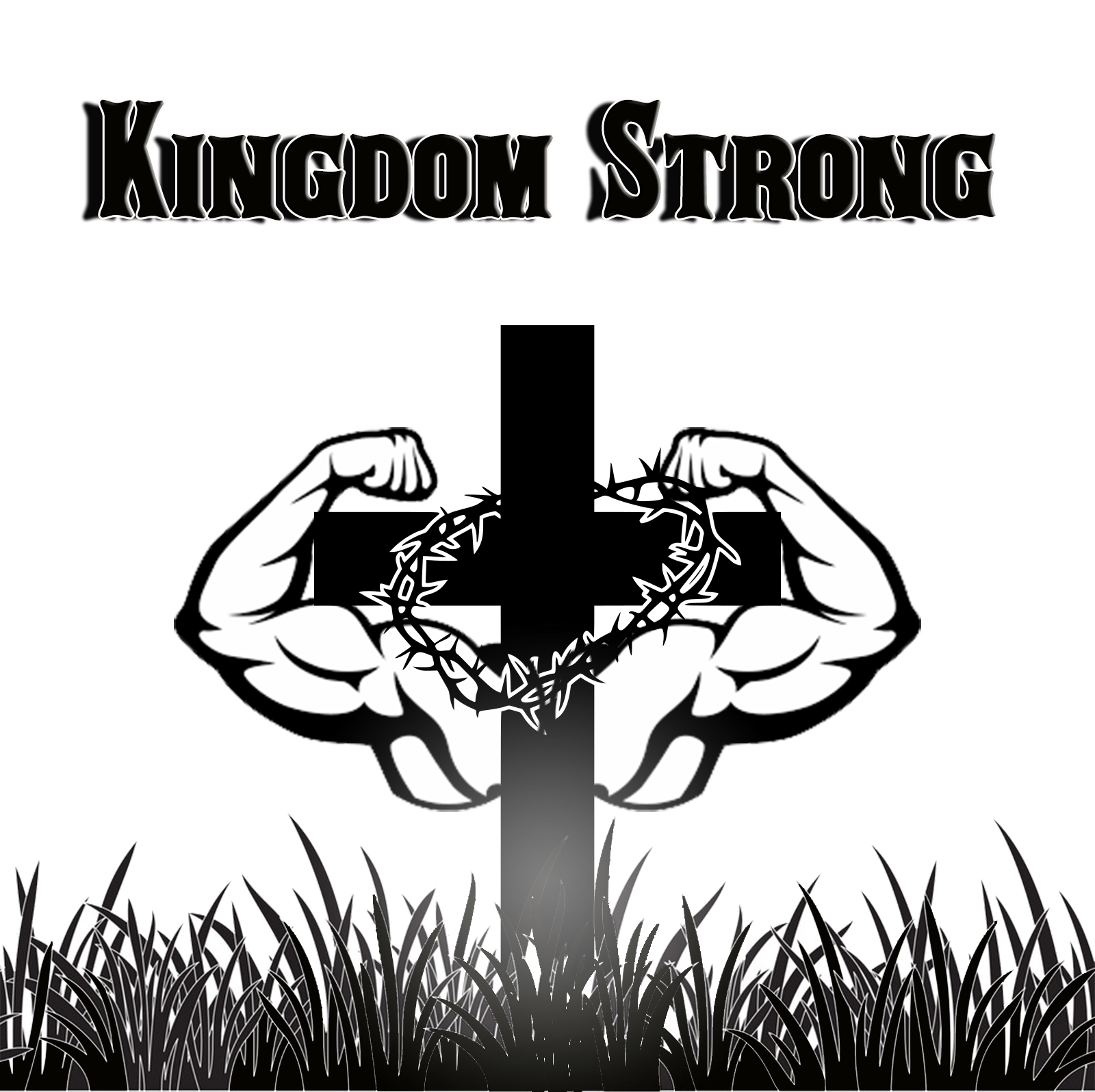The image is a large, square, black-and-white illustration. At the top, bold, three-dimensional black letters spell out "Kingdom Strong" with a subtle backdrop to enhance the 3D effect. Below this text, in the center of the image, stands a prominent black cross. Encircling the top of the cross is a crown of thorns, resembling barbed wire. From the middle of the cross, where the crosspiece meets the vertical post, emerge two highly muscular, white arms outlined in black. These arms curve upwards and form fists just above the horizontal T part of the cross. The powerful arms display well-defined shoulders, biceps, forearms, and hands, but no face or torso is visible. At the bottom of the image, a field of tall, black-shaded blades of grass stretches from left to right, reaching ankle height. The overall style of the image is animated, and it seems designed to inspire or attract attention, possibly as a poster for a fitness group or gym, or an album cover.